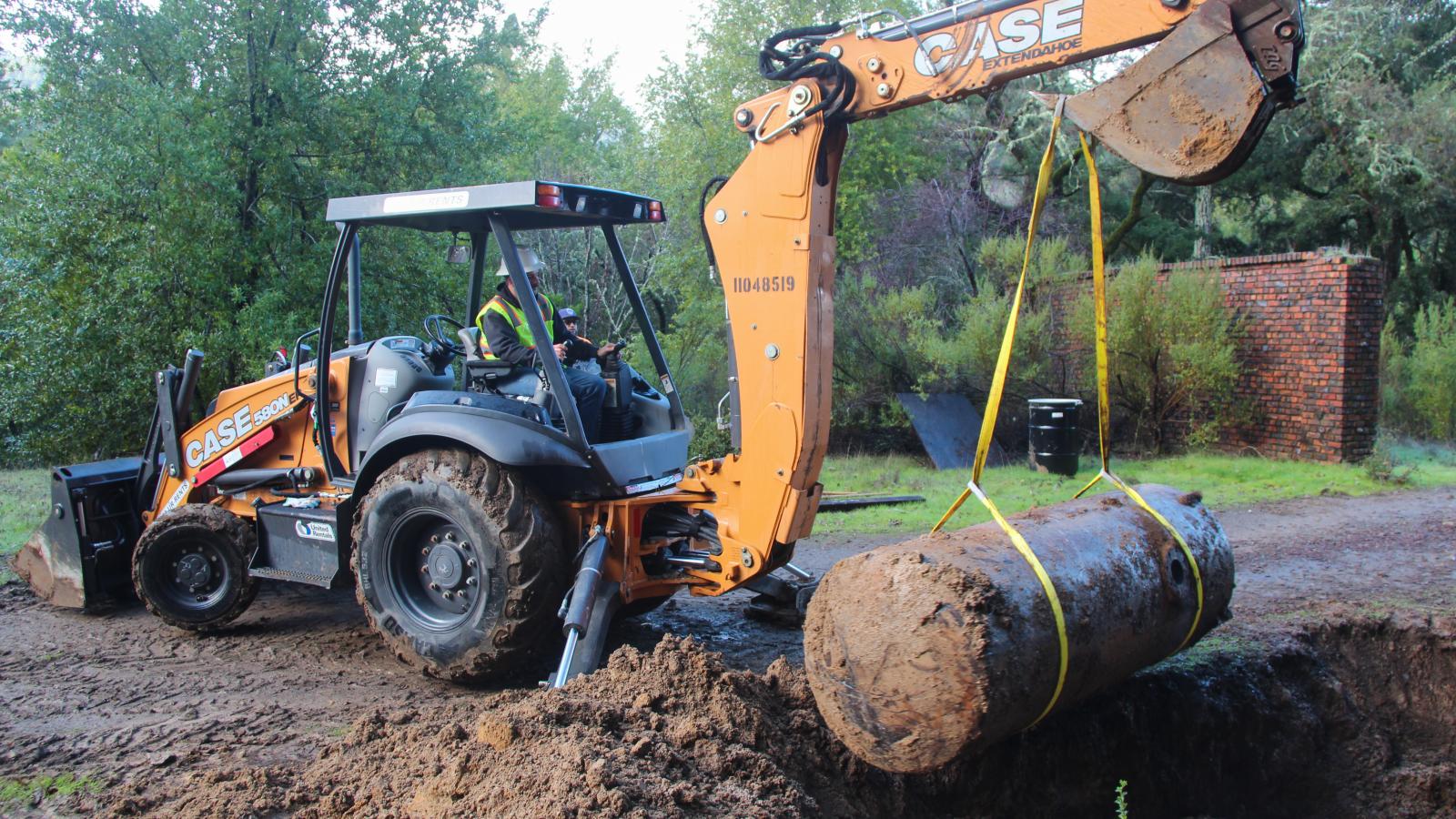The color photograph depicts a Case Extendohoe backhoe in a wooded area, actively lifting a large, cylindrical tank from the ground. The orange backhoe, with its bucket engaged and front wheels slightly elevated, showcases its digging and lifting capabilities. The tank, encrusted with dirt, is secured with yellow straps wrapped around it twice and is being hoisted by the backhoe’s bucket. A man in the operator's seat, wearing a white hard hat, jeans, a dark jacket, and a green and orange high-visibility vest, skillfully manages the machine. Another man stands nearby, offering assistance. The scene includes a small brick wall surrounded by trees and brush, indicating a rustic, outdoor setting. The backhoe's stability is ensured with its skids down, preparing for the heavy lifting task at hand.